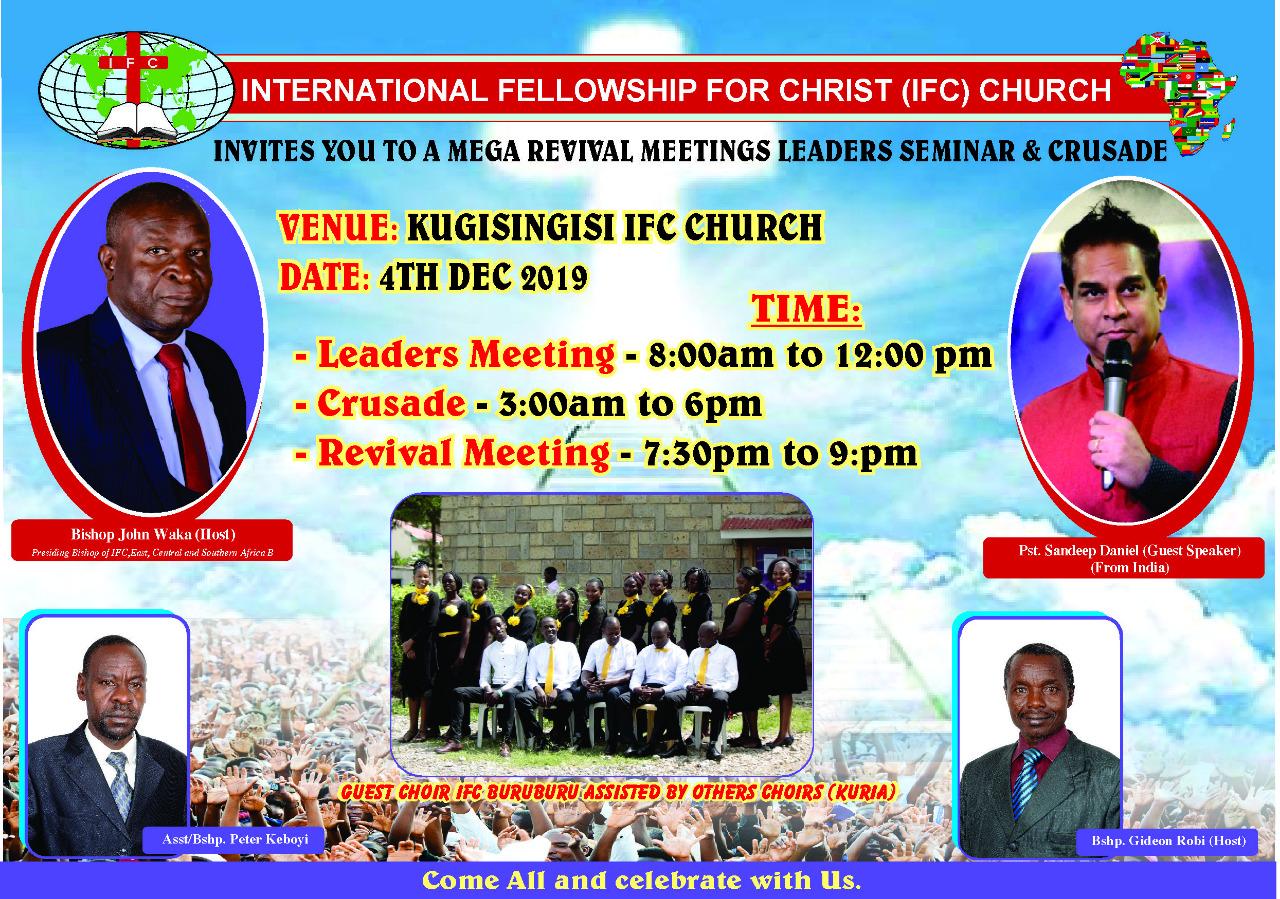This detailed poster advertises the International Fellowship for Christ (IFC) Church's mega revival meeting, Leaders Seminar, and Crusade, held on December 4th, 2019, at the Kuji Synod IFC Church. Set against a backdrop featuring a blue sky with white clouds forming a cross and snowy mountains, the poster prominently displays the IFC logo—a globe with green countries, a red cross, and an open book.

At the top, bold text reads "International Fellowship for Christ IFC Church," inviting attendees to the events. The schedule is clearly detailed: the Leaders Seminar from 8 AM to 12 PM, the Crusade from 3 AM to 6 PM, and the Revival Meeting from 7:30 PM to 9 PM.

The poster features photographs of four key speakers framed in red-bordered ovals. On the left is Bishop John Waka, a middle-aged black man in a black coat, white shirt, and red tie, who serves as the host and the providing bishop of IFC for East, Central, and Southern Africa. On the right is Pastor Sandeep Daniel from India, easily identified by his youthful appearance and microphone in hand. At the bottom left is Assistant Bishop Peter Kiboi, dressed in a black coat, gray tie, and white shirt. The bottom right features Bishop Gideon Roby, wearing a gray coat, maroon shirt, and blue striped tie.

Central to the poster is a group photo of the IFC Buruburu choir, assisted by other choirs, including Korea's. The image shows five black men seated in white shirts, yellow ties, and black pants, with twelve black women standing behind them, dressed in black with yellow scarves and flowers. This group is set against a background of a garden, a wall, and a notice board.

Anchoring the bottom is a blue strip with the welcoming words, "Come all and celebrate with us," and an image of a crowd with raised hands in celebration. The overall color scheme includes blue, yellow, black, and red lettering, contributing to the vibrant and inviting aesthetic of the poster.